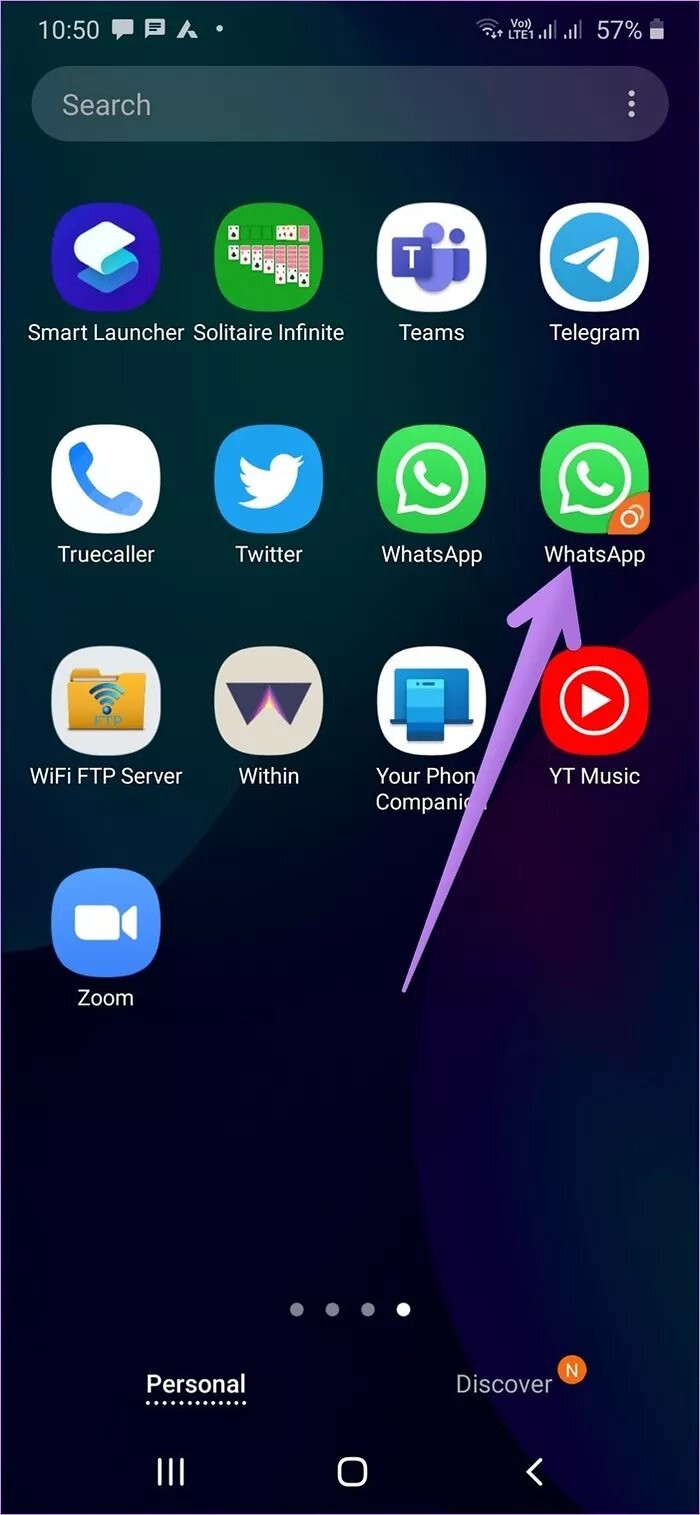A detailed screenshot of a smartphone homepage displaying a vibrant, gradient background in shades of dark blue, teal, and purple. At the top of the screen, white text and symbols indicate various notifications and statuses: the time reads 10:50, and the battery icon shows 57% charge. Additional icons display messages, Wi-Fi connectivity, and service bars. Below this, an opaque, rounded search bar with three white dots on the side and the word "search" in white letters is prominently featured. 

The main section showcases a neatly organized grid of application icons, with four rows. Each of the top three rows contains four apps, while the bottom row has only one. Notably, a large purple arrow directs attention to the fourth app in the second row, the green WhatsApp icon, which also bears a small orange corner, suggesting a notification. Other visible apps include Twitter, Teams, Telegram, Solitaire, Within, YT Music, Zoom, and Your Phone Company, each icon maintaining a rounded but slightly square aesthetic.